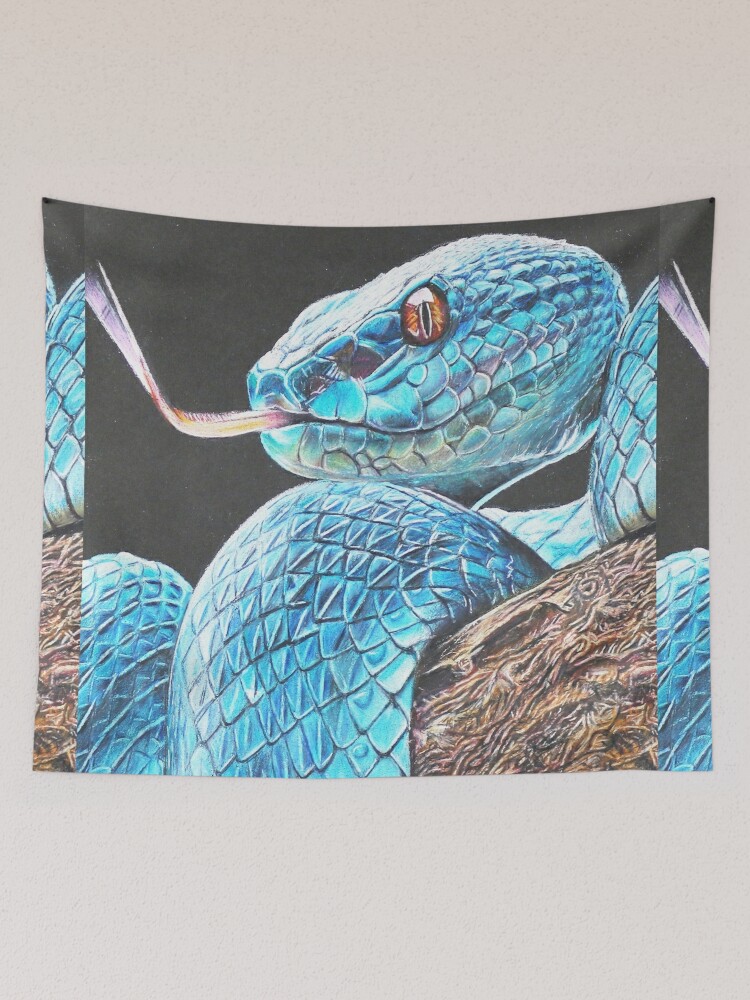In this portrait-mode image, we see a tapestry-like piece of fabric with a fuzzy texture, set against a light gray or beige background. The centerpiece is a stylized, aquamarine blue snake with accents of dark blue, light blue, and some hints of purple across its scales, giving it a pearlescent appearance. The snake is intricately wound multiple times around a brown tree branch, visible at the bottom right of the tapestry. The snake's head emerges at the top, facing towards the left, showcasing its brown eyes with narrow black slits and a long, pink tongue tinged with shades of lilac and pale orange. The backdrop of the snake itself is entirely black, contrasting with the light gray surroundings, making the blue hues of the snake stand out prominently. The detailed depiction captures the reflective quality of the scales, almost bringing the animated artwork to life.